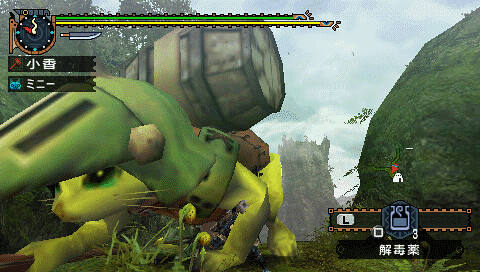The image is a detailed screenshot from a video game, featuring a zoomed-in view of the character on the front left side of the screen. The character appears to be a mouse or a yellow cat-like creature, crawling on all fours, wearing a green knight's helmet with the face-guard lifted. It is carrying a wooden barrel on its back. The background showcases a blue, cloudy sky and a cylindrical mountain to the right, with a green hill curving upwards towards the top right. Across the top of the image, two horizontal bars extend from left to right - the longer yellow bar and a shorter green bar, possibly indicating stamina or health. At the top left, there is a symbol resembling a knife and a dial or compass, with additional symbols including a hammer and a blue cat face, accompanied by Japanese characters. The bottom right displays a mini-map or score tracking graphic, also with three Japanese characters, indicative of position or lives remaining. The overall graphical style suggests it could be from an older console like the PS2 or GameCube.